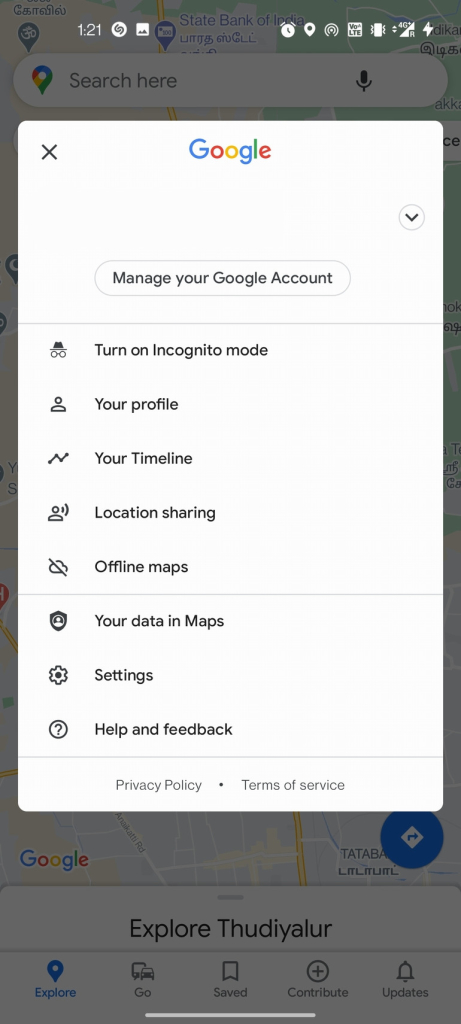This screenshot captures the interface of a popular mapping and navigation app on a smartphone, featuring several distinct elements. At the top of the screen, there's a Google search box accompanied by a pin icon for Google Maps. Below this, the text reads "Explore Sudiyarthudiyalur," indicating the area currently being viewed on the map. Users have the option to get directions from this location.

The app's navigation bar at the bottom of the screen displays five tabs: Explore (highlighted in blue), Go, Saved, Contribute, and Updates. The Explore tab is active and highlighted in blue.

Overlaying the map interface, there is a prominent section for managing the Google account, featuring:
- An "X" icon in the top left corner.
- The Google logo centered against a white background inside a gray circle.
- To the left of the logo, a drop-down arrow.
- Text stating "Manage your Google account" centered on a white background.

Below this, a horizontal line separates the account management section from a vertical menu offering various options:
- Turn on Incognito mode (illustrated by an icon of a disguised person).
- Your profile (represented by a stylized human figure).
- Your timeline (depicted by a rising graph icon).
- Location sharing (symbolized by a stylized person talking).
- Offline maps (shown with a cloud icon crossed out).

Another horizontal line separates these options from an additional vertical menu, indicating further functionalities within the app.